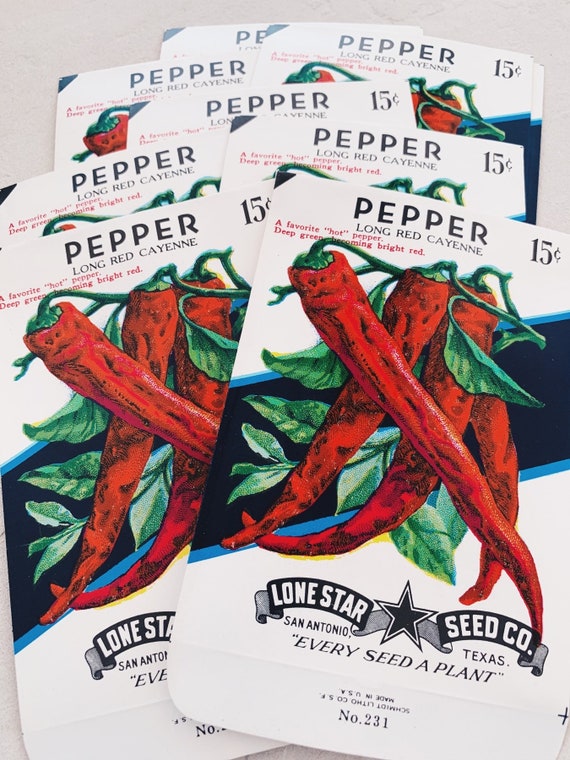Displayed are six packets of Lone Star Seed Company's 'Long Red Cayenne Pepper' seeds, each priced at 15 cents. The packets, predominantly white with a distinct blue stripe background, feature an image of long, thin cayenne peppers with green stems and leaves. Below the image, in black text, it reads "a favorite hot pepper, deep green becoming bright red." The top of the packet states "Pepper" in bold, black capitalized text, and to the bottom, a black banner with “Lone Star” on the left, “seed co” on the right, and a central black star framed by “every seed a plant,” San Antonio, Texas. The packets, seemingly from an era past, are laid across a white table with some overlapping, showcasing the unique, striking design of the packaging and the vivid red portrayal of the peppers.